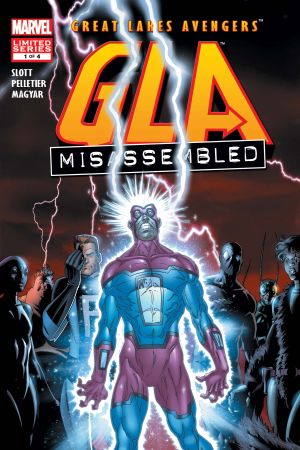This vertical rectangular frame resembles the cover of a Marvel comic book titled "Great Lakes Avengers." Dominating the lower half of the cover is a central, misshapen superhero figure in a translucent teal and purple bodysuit with a frog-shaped head and crooked fingers. The superhero bears a white rectangular emblem on his chest and sports purple gloves. Flanking this central figure are six other superheroes, each dressed in distinctive costumes and casting puzzled or concerned expressions towards him. To the left of the main figure stands another clear superhero figure with black gloves, wearing a black-and-blue costume. The backdrop of the cover features a dark, almost black sky with streaks of dark red. At the top, written in bright yellow and gold font, reads "Great Lakes Avengers" and "GLA." Beneath this, in white font, is the subtitle "Miss Assembled." The Marvel Limited Series logo is positioned in the upper left corner along with the names "Slot, Pelletier, Magia." The overall scene creates a dynamic and intriguing visual typical of comic book covers, hinting at a quirky and unconventional team of superheroes.